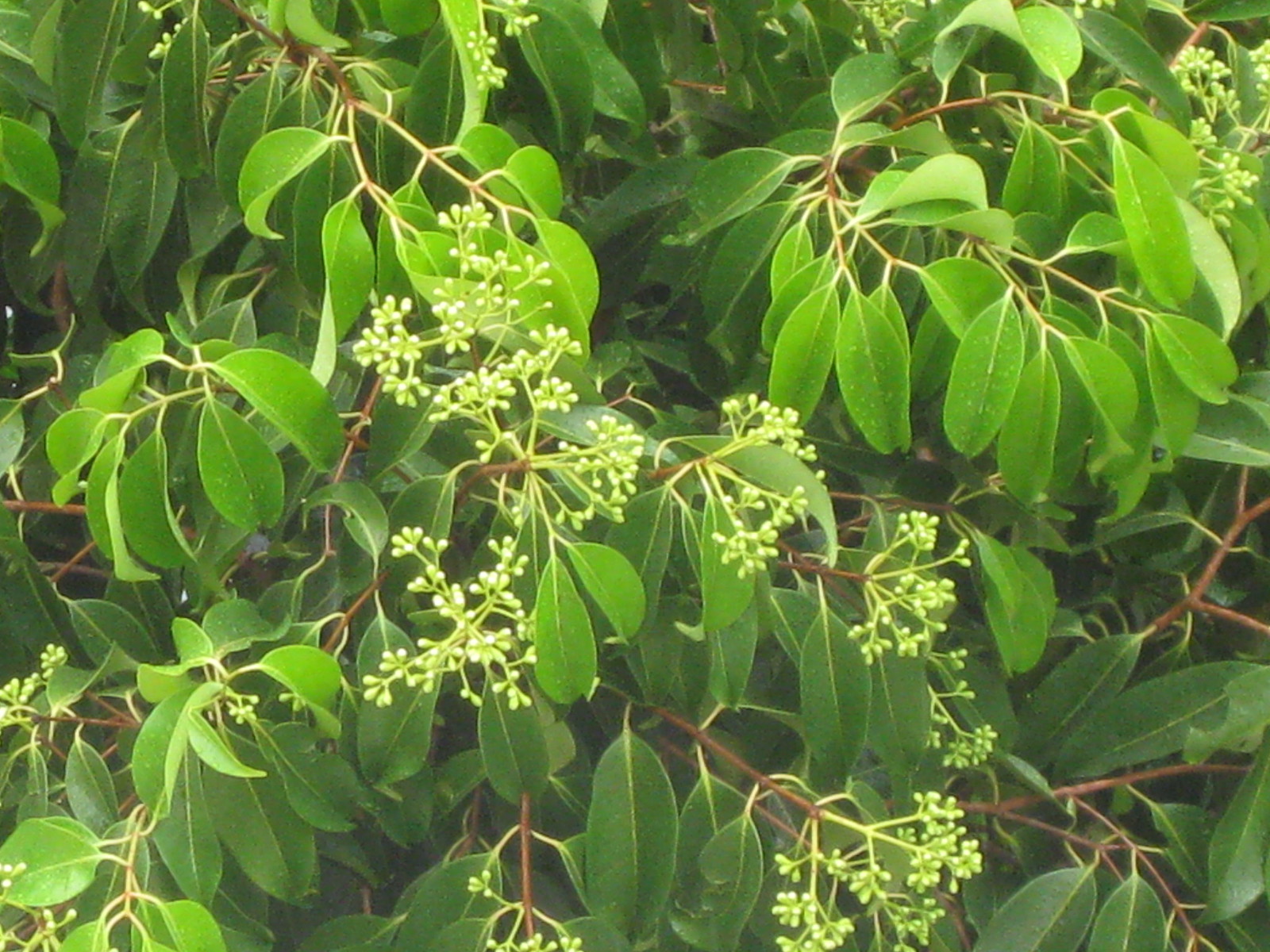The full-color daytime photograph showcases an outdoor scene featuring a lush, green tree canopy. The foliage consists of numerous large, banana-shaped leaves that are long and somewhat oval, hanging gracefully and densely in the air, creating a thick, leafy presence. The branches and stems are thin and brown, suggesting the tree might be young or it could even be a bush. Scattered among the leaves are delicate, white buds perched on very thin, extended stems, adding a touch of contrast to the verdant canopy. The scene appears vibrant and richly textured, hinting at a potentially aromatic environment.